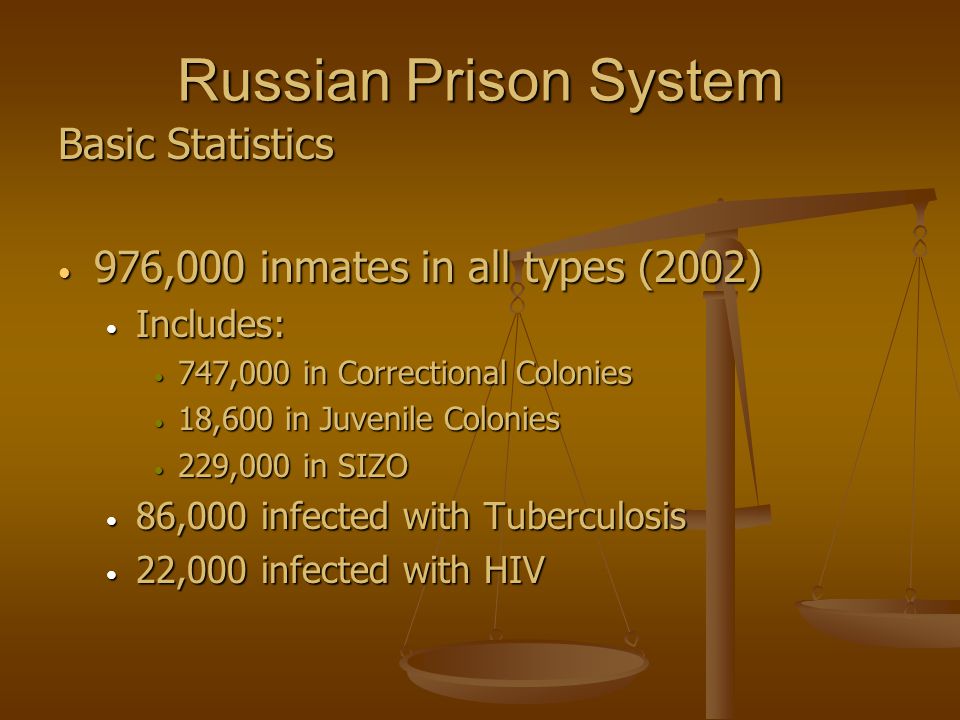The image presents an overview of the Russian prison system with detailed statistics, all set against a brown square background. This background transitions from a darker brown at the top and bottom to a lighter brown in the center. At the top center, the image is titled "Russian Prison System," followed by "Basic Statistics" aligned to the left. The text, in a light brown or pale yellow font, features four main bullet points: 

1. **976,000 inmates in all types (2002)**
   - Includes:
     - **747,000 in correctional colonies**
     - **18,600 in juvenile colonies**
     - **229,000 in SIZO (Pre-trial detention centers)**

2. **86,000 infected with tuberculosis**

3. **22,000 infected with HIV**

Additionally, the background of the image features the scales of justice, depicted in a medium brown color. The right scale tray is positioned higher than the left, adding a symbolic element to the visual representation.